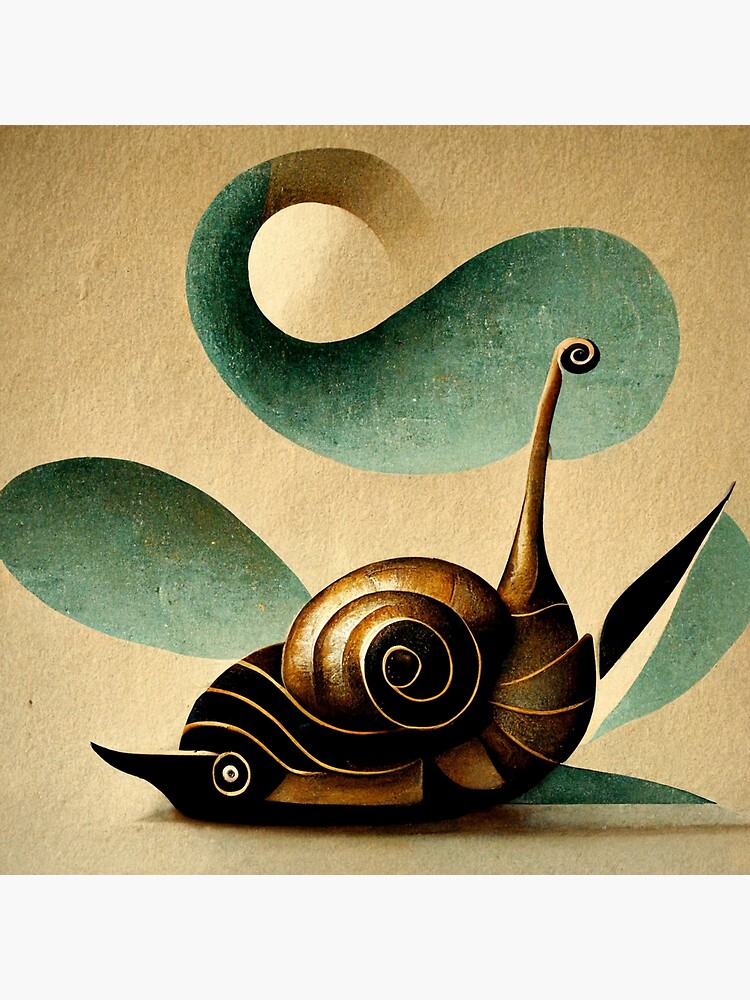This artwork features an abstract representation of a snail, prominently marked by a distinctive Fibonacci spiral for its shell. The snail’s body and shell are primarily brown with intricate golden stripes and thin black lines. The shell's lower left corner showcases a circular golden detail with a white dart and a black band around it. Rather than a traditional snail head, there is a whimsical curl extending from the narrow neck, adding an abstract twist. The background, which seems to be painted or drawn on a tan, textured surface resembling handmade paper, includes various green shapes; one at the top that subtly resembles a whale without fins, and another resembling a leaf to the right of the snail. The green shapes add a leafy, natural atmosphere to the scene, complementing the earthy tones of the snail and evoking the imagery of a verdant environment. The overall piece has a square format, and its textured appearance suggests it might be painted on a wall, providing a unique, almost optical-illusion-esque visual experience.